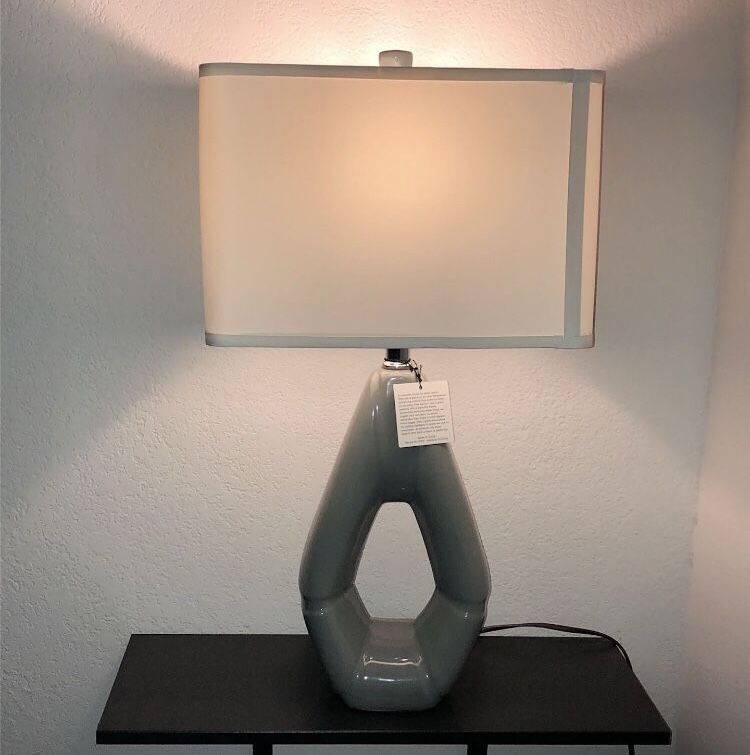The image depicts a small, dark grey rectangular desk positioned against a plain white wall. On the desk sits a modern and somewhat abstract lamp, emitting a warm, amber light. The lamp has a unique design with a white rectangular shade framed in grey on the top, bottom, and right side. The base of the lamp is pentagon-shaped with an elongated upper section and features a conspicuous cutout in the center. Made from shiny grey material, the base adds a distinctive touch to the lamp’s overall appearance. Hanging just below the shade is a tag with some unreadable text. The lamp's power cable is visible trailing to the bottom right corner. Overall, the lamp’s artistic design stands out, making it a focal point in the otherwise simple setting.